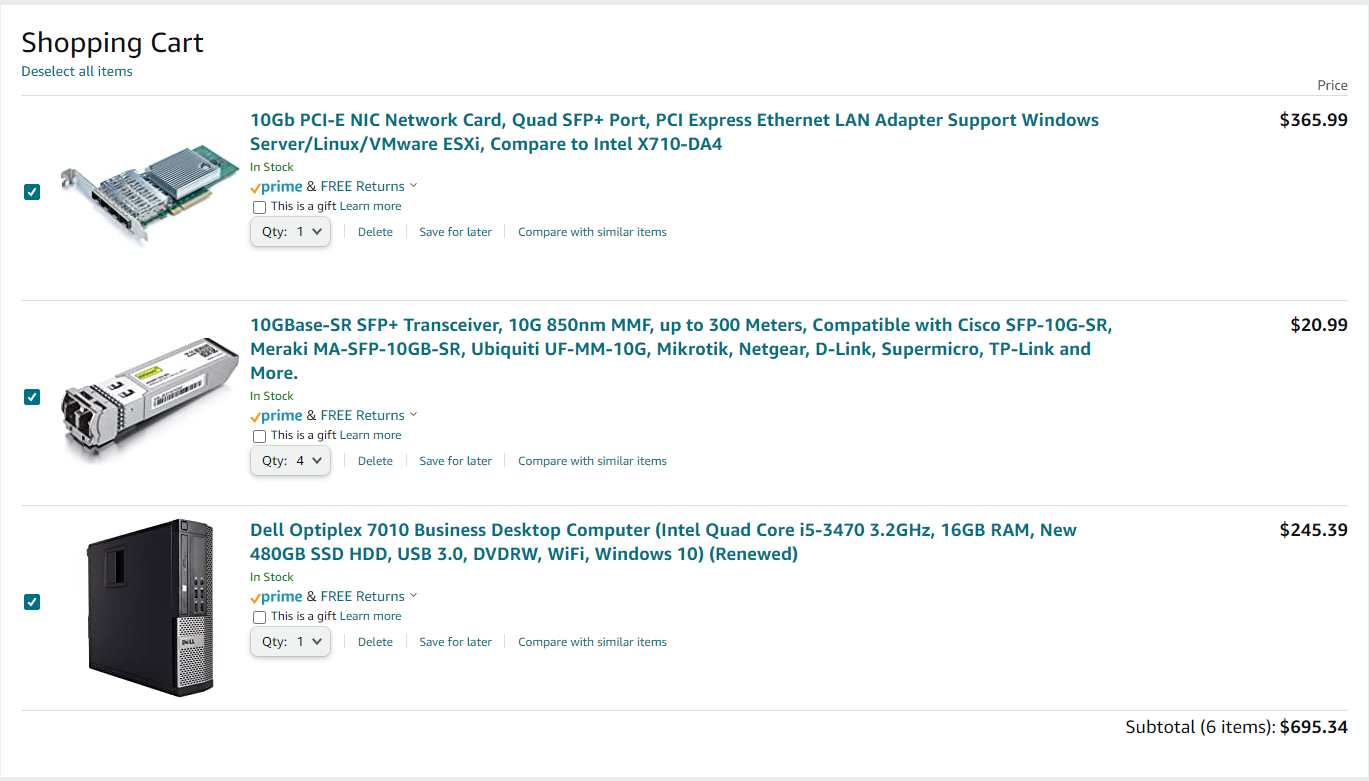This image captures an online shopping cart filled with various computer parts. The interface offers an option to deselect all items and features checkboxes to the left of each item for individual selection. The cart includes the following:

1. An Ethernet cable priced at $365.99.
2. A TP-Link connection device, which is compatible with Cisco, priced at $20.99. This item resembles a small, silver connector and is described as a base.
3. A Dell business desktop computer, fully depicted, priced at $249.39.

Additionally, the cart contains four more connection devices; however, they are not individually detailed. The subtotal for all six items (one Ethernet cable, one TP-Link connection device, one Dell desktop computer, and four other connection devices) is calculated at $695.34, displayed at the bottom of the shopping cart. Note that the subtotal does not yet include tax or shipping fees.